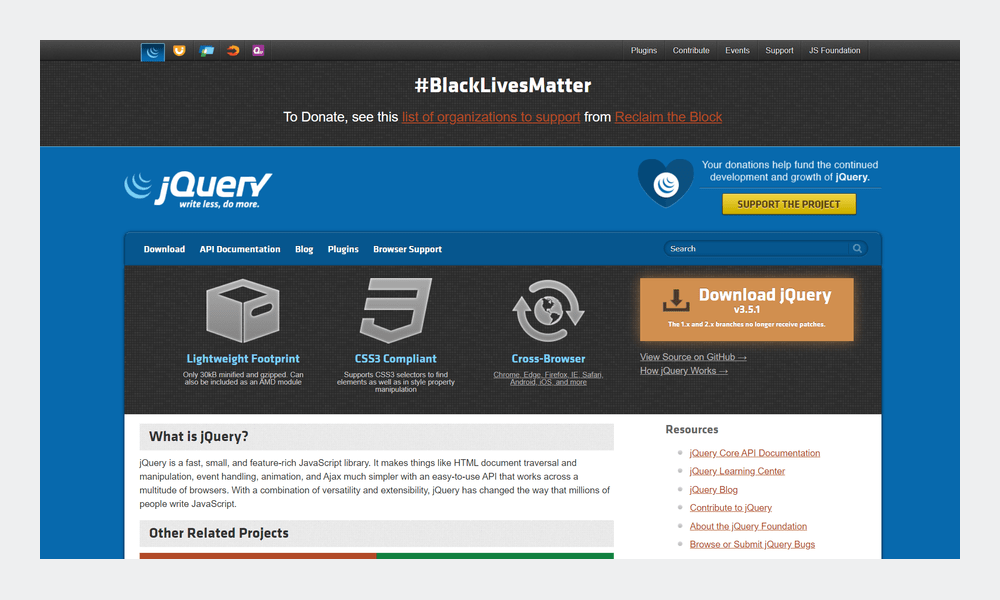The image depicts a screenshot of a website, featuring a prominent banner at the top with a black background, displaying the hashtag "#BlackLivesMatter." Below this message, the banner encourages visitors to support the movement by donating to listed organizations from Reclaim the Block, likely in response to a significant event.

The main section of the website follows the banner and showcases a professional and clean layout with a color scheme of blue, gray, and white. At the top left corner, the site is branded with the name "jQuery" accompanied by the slogan "Write Less, Do More."

On the right side, there is a message encouraging donations to support the ongoing development and growth of jQuery. Below this message is a prominent yellow button labeled "Support the Project."

The website features a set of navigational tabs and a search bar. The tabs include options for "Download," "API Documentation," "Blog," "Plugins," and "Browser Support." Adjacent to these tabs is the search bar for user convenience.

The main content of the page appears to be focused on downloading jQuery. A large, vibrant orange button invites users to "Download jQuery Version 3.5.1." Beneath this button, there is a note indicating that the 1.x and 2.x branches no longer receive patches.

Additionally, the page includes detailed descriptions and links to further information about jQuery, associated projects, and available resources, with hyperlinks highlighted in orange for easy navigation.